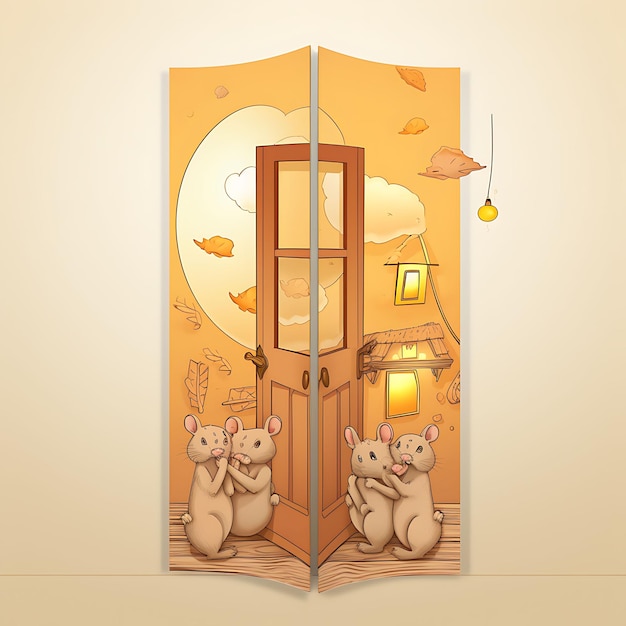The artwork consists of two paintings displayed on a pale beige wall, both uniquely shaped with arc-like curves, creating trapezoidal forms that meet when aligned. These predominantly yellow pieces together form a cohesive image that centers around a wooden door. Each painting features a scene involving two beige mice with pink ears, depicted on either side of the door, standing on a wooden floor. The left panel presents the mice beneath a window that streams in light, surrounded by floating orange and brown leaves and a yellow circle resembling the sun. The right panel mirrors this setup with the mice standing near the door under a light bulb hanging from a string, also amidst the same ambient details of floating leaves and ethereal light. The imagery suggests a narrative where the mice seem to be hiding or interacting with their surroundings, evoking a whimsical and cohesive tableau when viewed together.